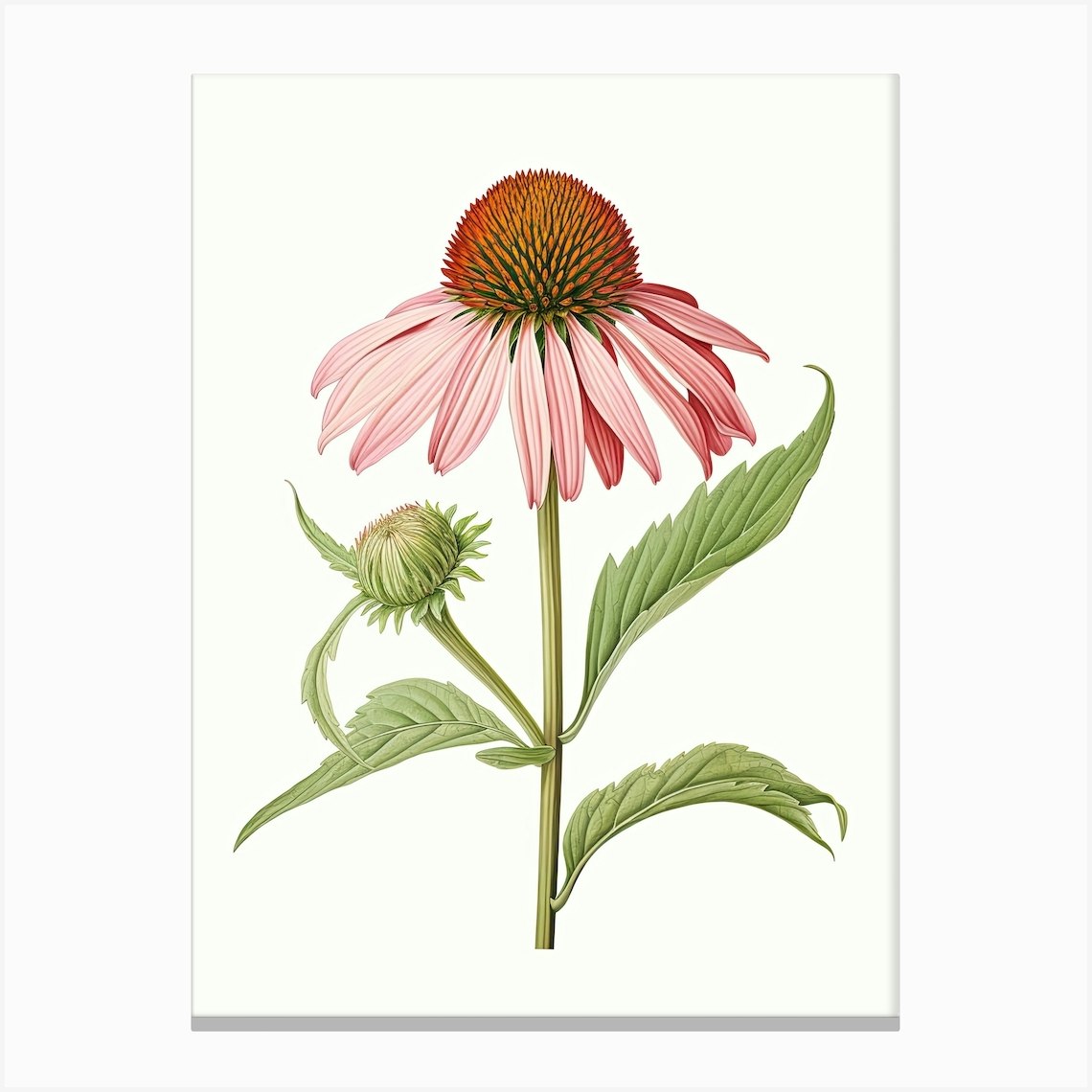This image depicts a delicate, colored pencil drawing of a daisy-like flower set against a white background. The flower's light green stem supports three equally green leaves and a budding flower that has not yet bloomed. At the top of the stem, a fully bloomed flower showcases numerous oval-shaped, pointed petals that are a soft pink, gently arching downward. The center of this flower features an intricate mix of colors, with rich, prickly textures in greenish, reddish, and pinkish hues, adding depth to its appearance.